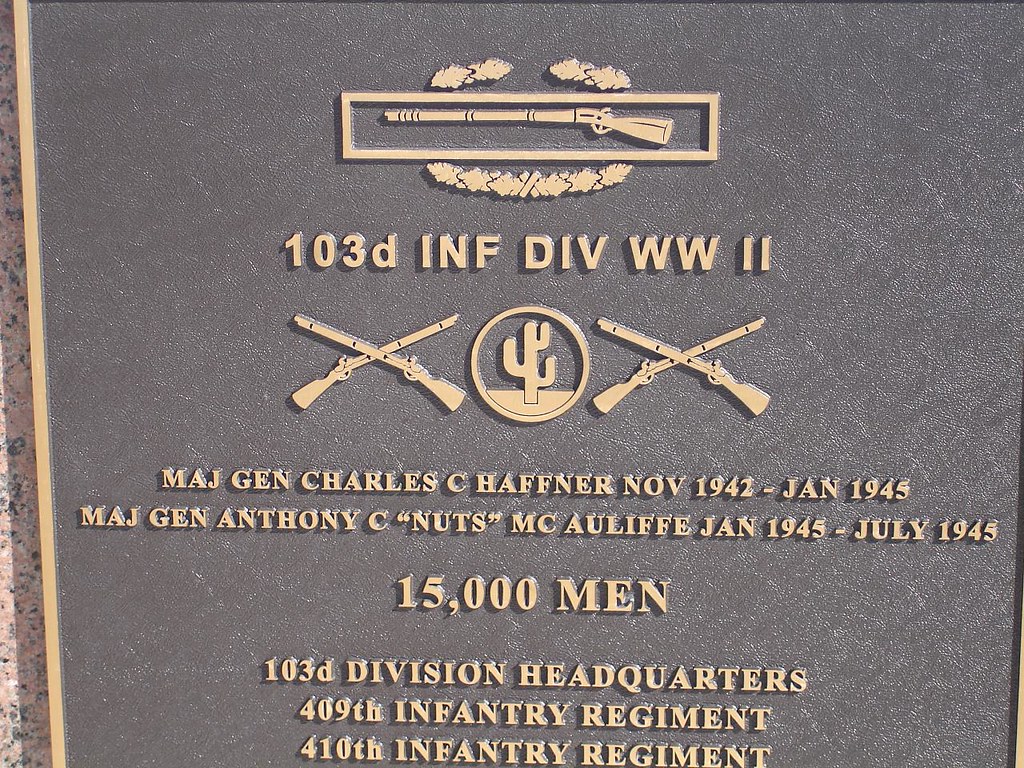This image features a close-up of a historical memorial plaque, mounted on a stone wall. The plaque has a black background with a gold border. At the top, there is a rectangle enclosing a rifle with decorative elements surrounding it. Below this, the inscription "103D INF DIV WW2" is prominently displayed. Further down, a cactus encapsulated within a circle is flanked on either side by crossed rifles forming an X shape. The text reads: "Major General Charles C. Hafner, November 1942 to January 1945" followed by "Major General Anthony C. 'Nuts' McAuliffe, January 1945 to July 1945." The plaque concludes with details about the division, noting "15,000 men, 103rd Division Headquarters, 409th Infantry Regiment, 410th Infantry Regiment."